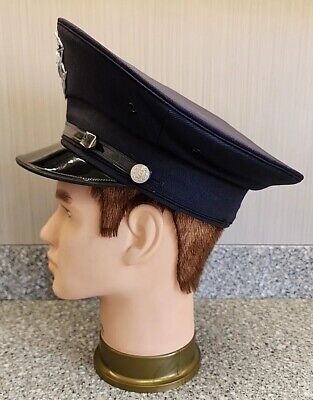This is a detailed photo of a mannequin's head positioned from the neck up, resting on a speckled gray countertop. The mannequin’s skin is white, with a short brown wig styled into a neat haircut. Around its neck, there's a gold or brass-colored section that serves as a base. In the background, a white wall with subtle gray lines enhances the neutrally toned setting.

The head is oriented to the left, showcasing the mannequin's profile which includes dark eyebrows and a detailed face reminiscent of a white Caucasian male. Atop the head, it sports a dark blue police hat with a shiny black bill. The hat features a silver badge on its front, a black leather strap with a silver buckle, and a matching detail on the side securing the buckle. This combination of accessories suggests an official police headgear, accentuating the uniformed appearance of the mannequin.